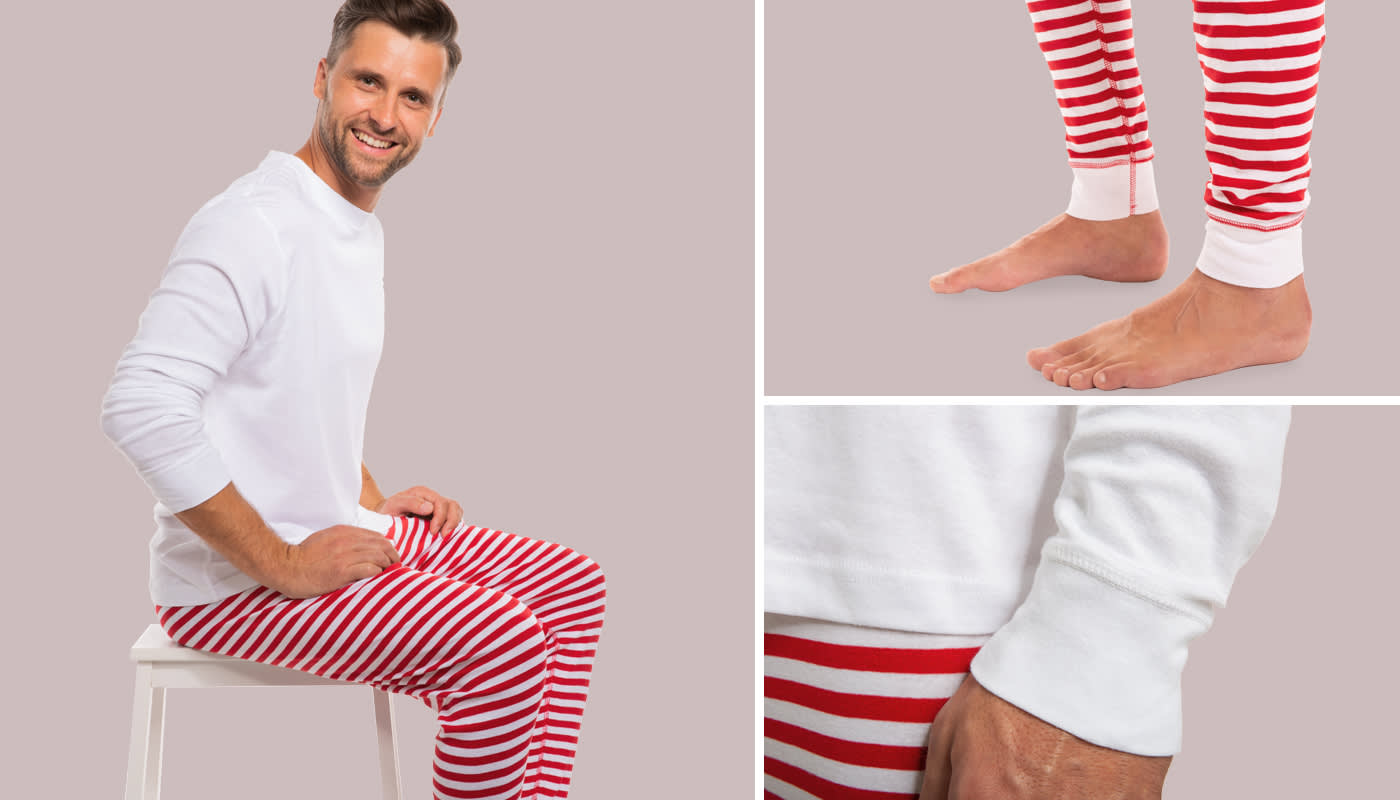A composite image showcases a white man with brown hair and a trim beard, seated on a white stool against a pinkish-gray backdrop. The main figure, positioned on the left, sports a broad smile as he models a distinctive outfit. He is clad in a long-sleeved white shirt, the sleeves casually rolled up to his mid-forearm, and striking red and white horizontal-striped pants, which are cropped at the lower leg, revealing no feet. His attire evokes a whimsical candy cane-like appearance. 

The upper right close-up zooms in on the lower portion of the pants and his bare feet, emphasizing the white cuffs against the pinkish-gray wall. The bottom right image provides a detailed view of his white shirt with the sleeves rolled down to the wrists, showcasing the cuffs and a glimpse of the red and white striped pants. The aggregate of these images captures the quaint and playful essence of the outfit, reflecting a harmonious blend of casual ease and vibrant design.